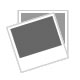The image depicts a vintage Paragon Needlecraft embroidery kit sealed in a clear plastic bag. The standout feature within this package is a delicate white baby dress, likely intended for christening, prominently displayed in black and white. The top and bottom edges around the collar and hem appear designed for hand embroidery. The packaging includes several noteworthy labels: "Paragon Needlecraft" is written in white on a pink background, while black text declares it to be a "stamped quality sanitized Nansuk baby Gertrude for embroidery." Further information reveals that "This Gertrude is fashioned after the finest ready-made baby wear," and it comes "Amplify cut, clean-seamed, ready for delicate touches of embroidery with para lustra file art 216 strand embroidery thread." Also included are detailed instructions for embroidery, recommending Paragon Needlecraft lace number 647, imported from France, for trimming. The package and product combine to reflect a bygone era of detailed handcraft and personalized baby garment creation.